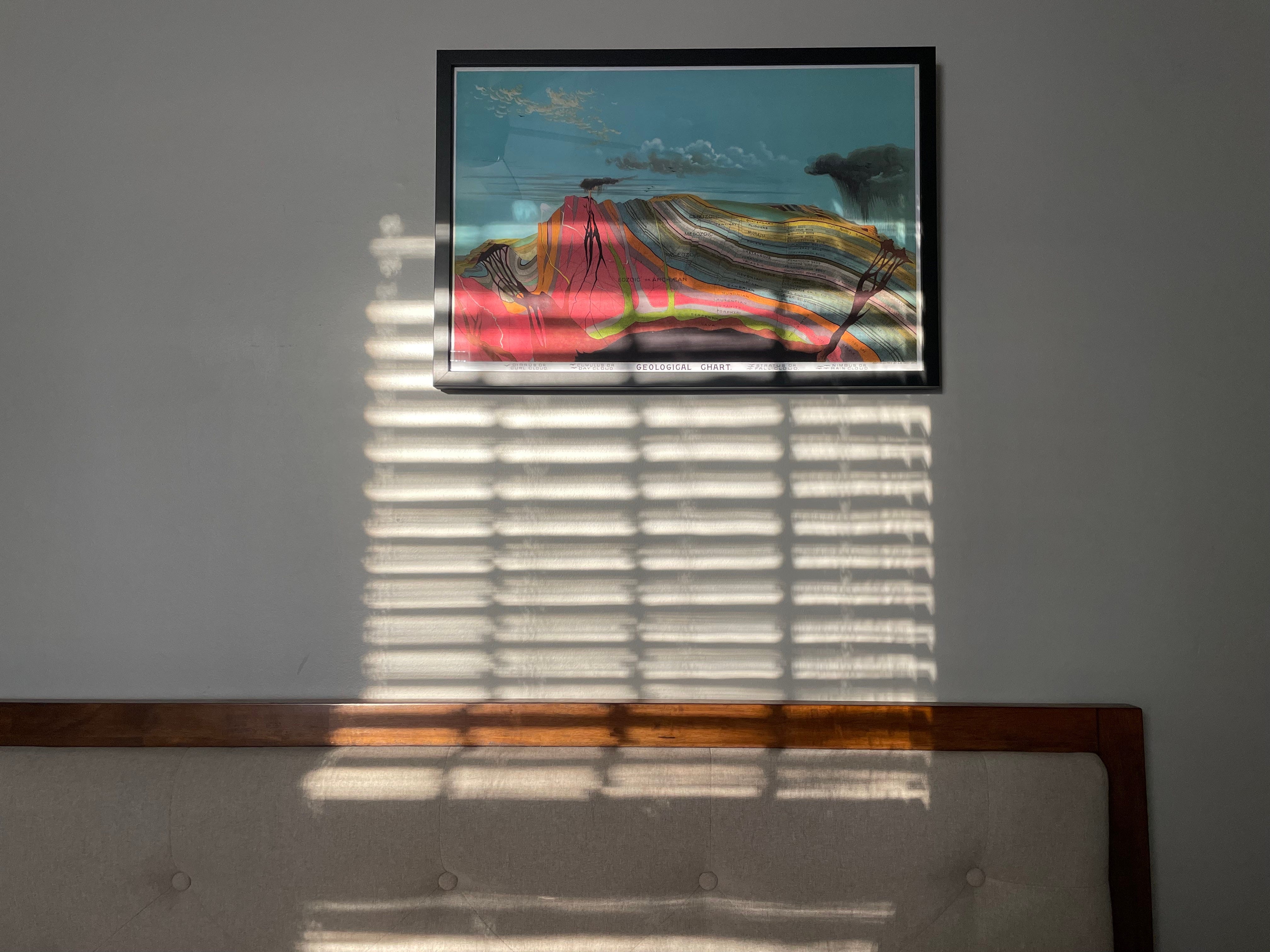The image showcases a serene bedroom scene with a detailed focus on the lower third. Dominating this portion is a tufted gray headboard, accentuated by a wooden frame in a rich brown hue. Clearly visible on the headboard are buttons that add a touch of elegance. Mounted above the headboard is a captivating painting with a distinctly Japanese-inspired aesthetic. It features a figure in a vibrant red and intricately patterned garment that blends harmoniously with the surrounding scenery—suggestions of mountains, trees, and a serene blue sky created in a watercolor style. Below the painting, blurred lettering adds a traditional touch, all encased in a simple, thin black frame. A window situated opposite the bed allows sunlight to stream in, casting shadows of window shades across the upper portion of the bed and the lower part of the painting, with the shades' patterns vividly imprinted by the sun's intense glare.